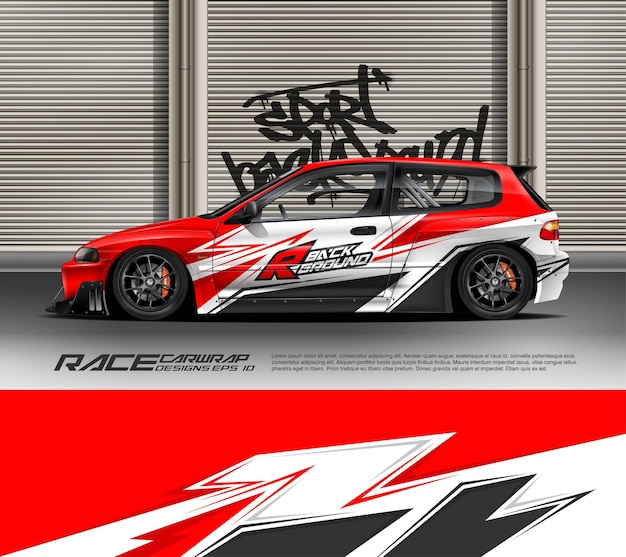The image is a detailed render of a race car set against a cartoonish backdrop of a garage with graffiti. The car, predominantly red and white with touches of black at the bottom, is oriented so that its front is pointing to the left. On the center of the door, the text "R Background" is prominently displayed. Just below the car, there’s another piece of text reading "Race Car Wrap Designs EPS-10". The background features graffiti, which appears to spell out "Sport Background". Additionally, there is a logo near the bottom that bears resemblance to the one on the car, though slightly different. The style of the image is illustrative rather than photorealistic, emphasizing a graphical quality ideal for display.